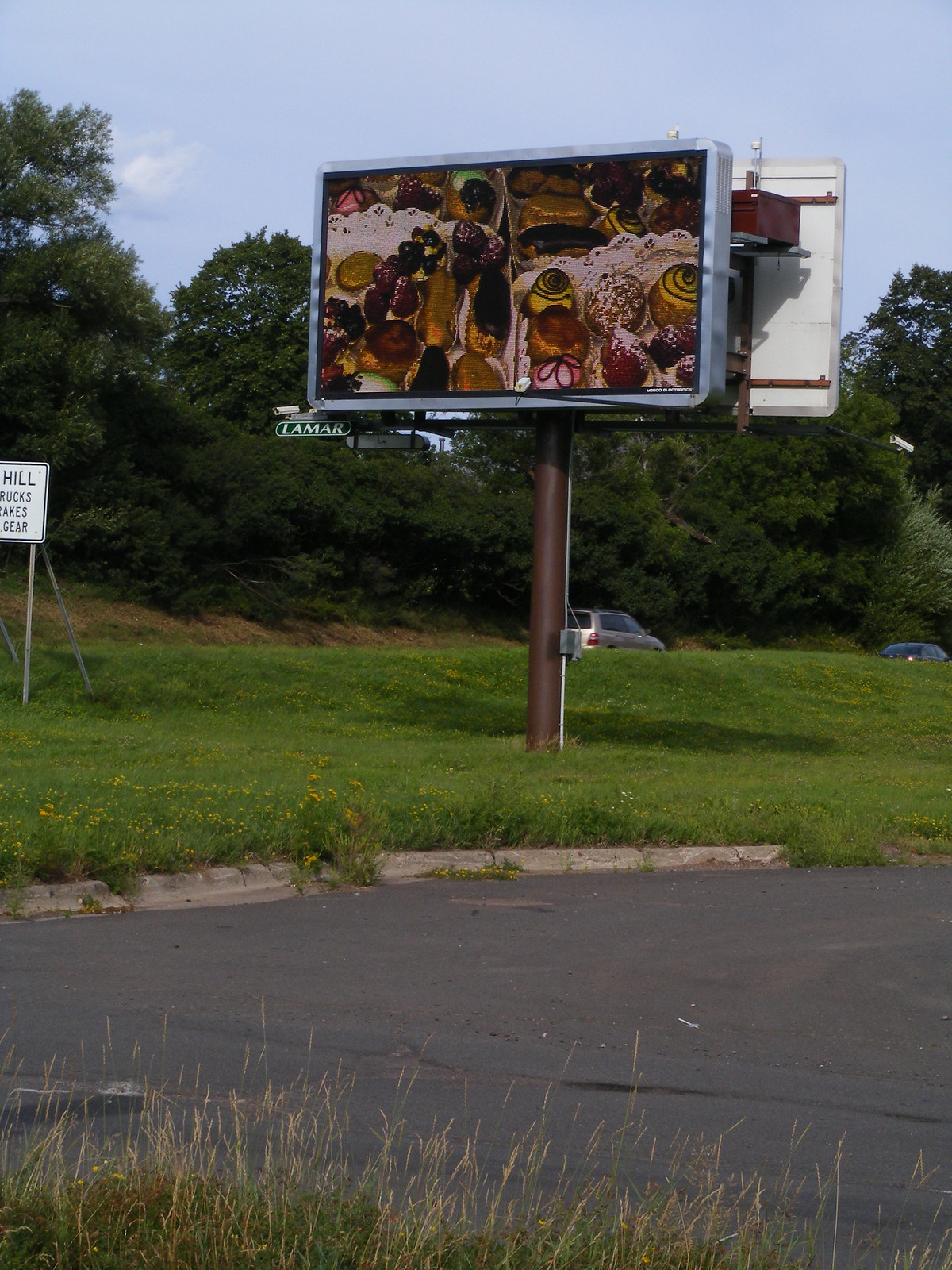This outdoor daytime colour photograph in portrait orientation prominently features a digital billboard situated on a grass median beside a roadway, flanked by a car park. The billboard displays an intricate graphic image of assorted pastries and chocolate bonbons on frilly white doilies, suggesting an advertisement for a local pastry store, although no text is present to confirm this. The delectable treats include chocolate confections with green icing and chocolate swirls, powdered sugar-dusted chocolates, pink-iced pastries with brown chocolate blossoms, and possibly glazed chocolate and maple-flavored bar-shaped doughnuts. The billboard is mounted on a thick, circular, vertical pole emerging from the grass. In the background, a silver station wagon and a black sedan are visible, with one car driving to the right. The parking lot in the foreground features dark grey asphalt bordered by stone grey and white-colored kerbstones and is surrounded by slightly overgrown grass. Trees with green foliage can be seen on a small hill beyond the road, adding a natural backdrop to the scene. Additionally, a white sign with unreadable black text is present along the road.